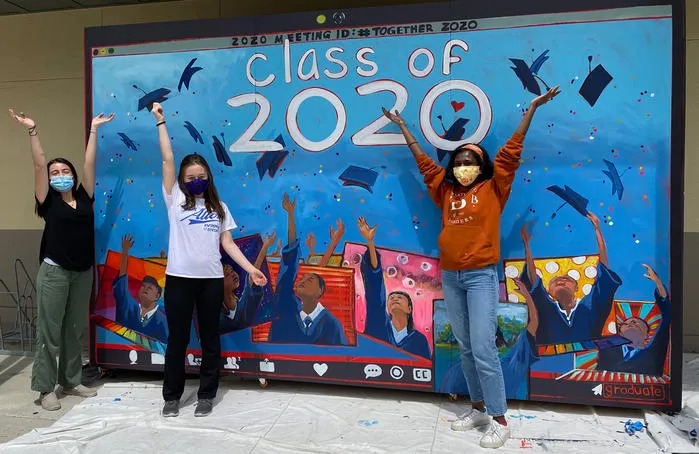In this vibrant and celebratory scene, three young ladies stand proudly in front of a large mural that commemorates their graduation year, 2020. The mural, painted with a captivating mix of light and medium blues, features bold black lettering at the top reading "ID hashtag together 2020". It depicts joyous students in blue graduation robes, energetically throwing their caps into the air amidst an explosion of colorful confetti. Each student in the mural is portrayed within a uniquely designed background—ranging from yellow with white polka dots to shades of pink with black and white polka dots, and even orange hues.

Standing before this lively artwork, the three girls—two white and one black—exude happiness and a sense of accomplishment. Two of them have both arms raised jubilantly, while the third raises one arm high. All three wear masks, hinting at the time during the COVID-19 pandemic. The floor beneath them is covered with a drop cloth, splattered with paint, suggesting they just completed this artistic tribute to their graduation. Their joyful postures, despite the masks, reflect the excitement and unity of their class, celebrating their achievements together indoors.